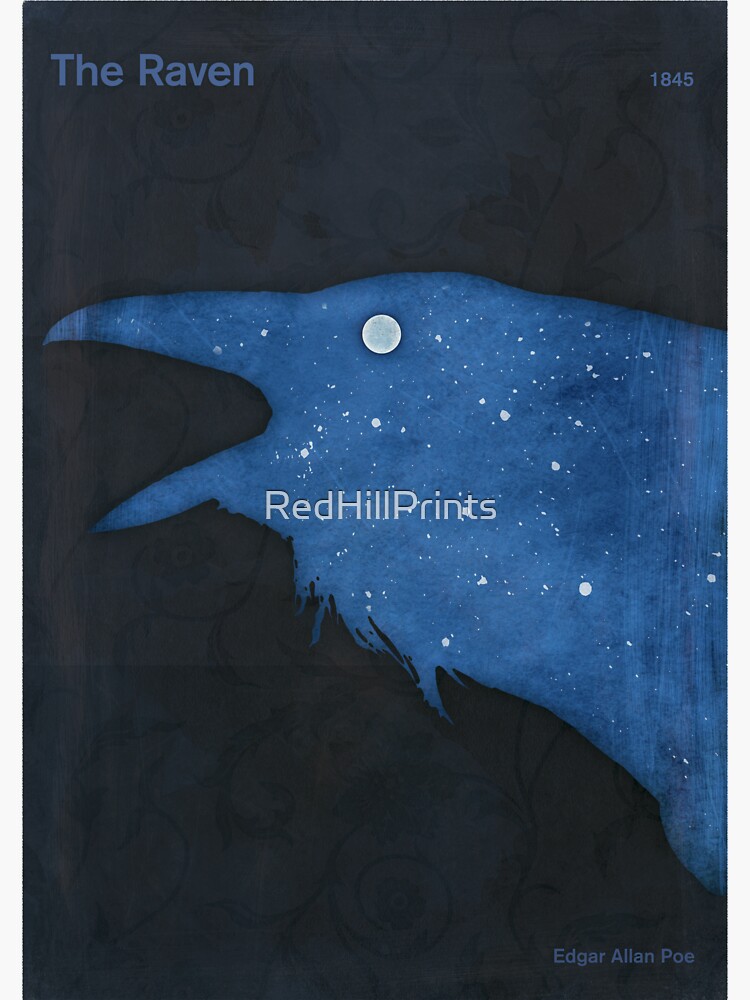This rectangular image, taller than it is wide, features a predominantly black background with notable text and illustrations. At the top left corner, in blue writing, it reads "The Raven," while the top right corner marked with the year "1845" signifies the era associated with the artwork. Dominating the center is an ethereal outline of a raven, depicted in dark blue like a night sky, adorned with white specks resembling stars. The raven's beak points towards the left edge of the image, and its eye, which is represented by a lifelike moon, adds to the celestial theme. Across the raven’s body, written in white text, is "Red Hill Prince." Additionally, a small signature at the bottom left corner indicates the artist's name, "Edgar Allan Poe," rounding off this visually striking piece with literary reference.